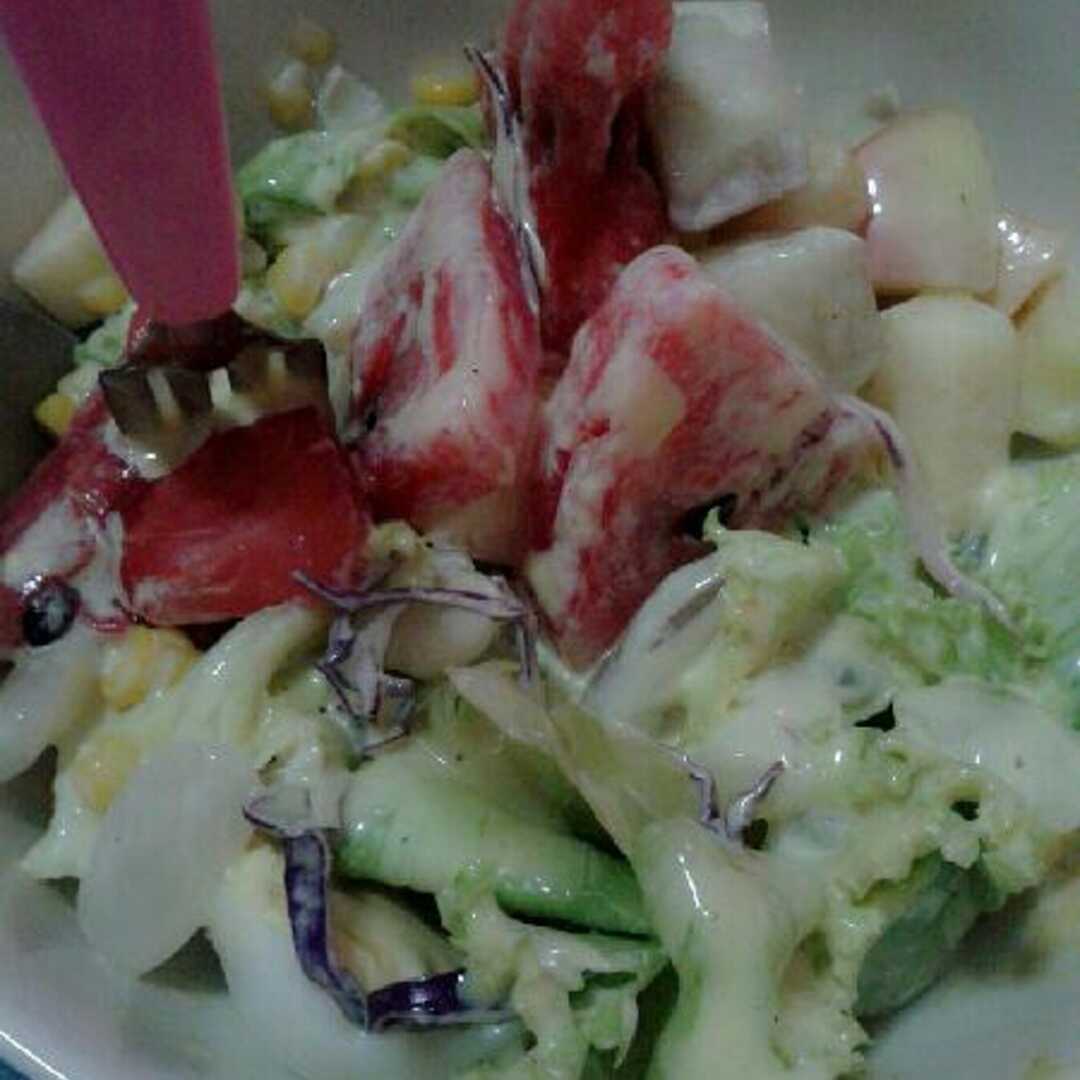This close-up image features a vibrant and colorful salad, likely a fruit salad adorned with a creamy, white dressing. Centered in a white bowl or plate, the salad boasts a variety of fruits and vegetables, vividly bright and appealing. On the left-hand side, a fork with a pink handle is visibly stabbing into a red chunk, possibly watermelon or strawberry. The composition includes square pink objects that might be radishes or watermelon, purple cabbage strands, and white squares that resemble cut-up apples. Scattered throughout the salad are hints of other fruits and vegetables like green cucumber slices, kernels of yellow corn, and possibly mashed green grapes. The entire mixture is enveloped in a glossy, white or clear dressing, creating a deliciously inviting appearance. The setting of this close-up shot could be in a kitchen, a restaurant, or even intended for a food blog, emphasizing the appetizing diversity of the salad ingredients.